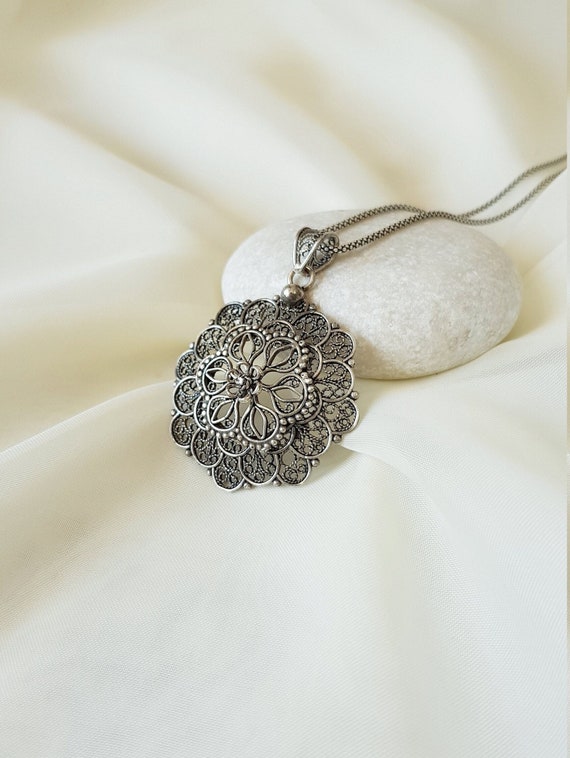The photograph captures a meticulously staged product shot intended for print or online use, showcasing an ornate pendant necklace. The pendant, a flower-like design crafted from dark silver metal that appears slightly tarnished, exhibits a circular shape made up of smaller, petal-like circles. It features five prominent segments—one central and four radiating outward—reminiscent of intricate ironwork. The necklace is elegantly draped over a smooth, round, white stone, which is slightly larger than the pendant itself. This composition is set against a billowy, creamy white fabric that exhibits subtle indentations and ripples, adding texture to the background. The overall presentation suggests an antique yet valuable piece, highlighted by the photograph's detailed and decorative styling.